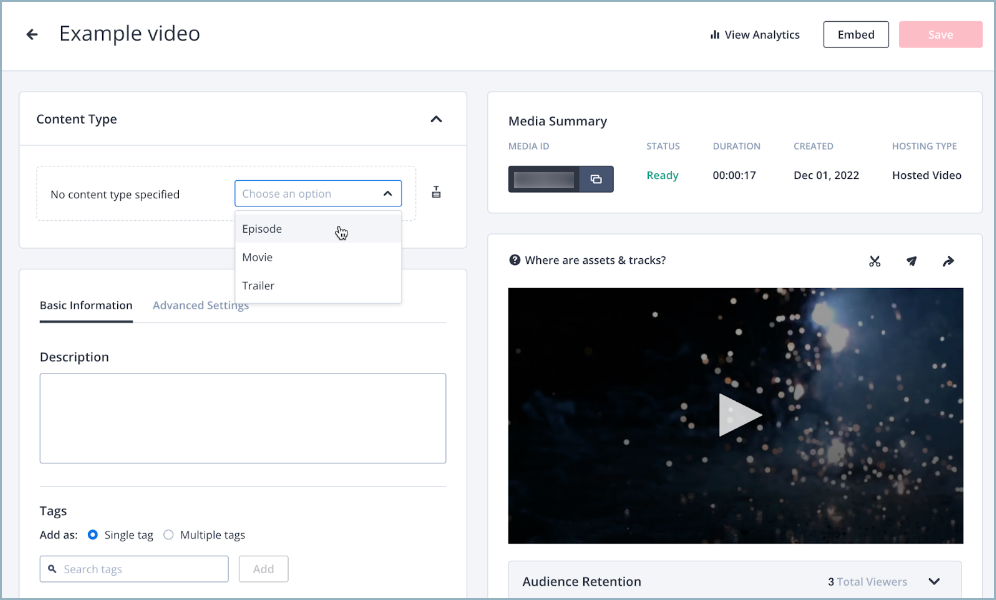This image is a screenshot from an analytics website, showcasing an example video tutorial on how to use the website. The video content type hasn't been specified yet, but options available include "Episode," "Movie," and "Trailer." Below these, there is a section to provide a basic description, which remains empty for now but can be filled in later. Additionally, there is an option to add tags to the video.

In the bottom-right corner of the screen, there is a feature to view and track the assets associated with the video. The uploaded video, possibly the media type specified earlier, currently has three total views, as indicated by the audience retention bar.

Details provided show that the video was created on December 1st, is hosted, and has a duration of approximately 17 seconds. The status of the video is marked as "ready." Other than these details, the screen does not display any additional information.